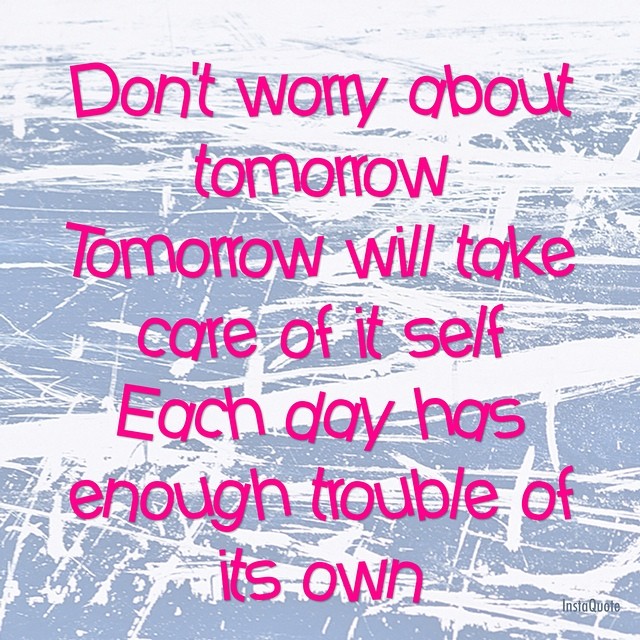The image is a square piece of abstract artwork featuring a rough, scratched blue and white background that appears splattered and scribbled upon, creating an uneven and rustic texture. The background transitions from primarily white at the top to a light bluish-gray with more spread-out white splatters toward the bottom, intersected by a prominent long white line running diagonally across. Over this background, a motivational quote is displayed in bright pink, cartoonish and slightly zig-zaggy text that reads, "Don't worry about tomorrow. Tomorrow will take care of itself. Each day has enough trouble of its own." The text appears scattered, with letters at different angles, featuring mismatched spacing, adding to the whimsical and non-uniform aesthetic. In the bottom right corner, the word "INSTAQUOTE" is printed in tiny grayish-green font, further adding to the artistic style of the piece.